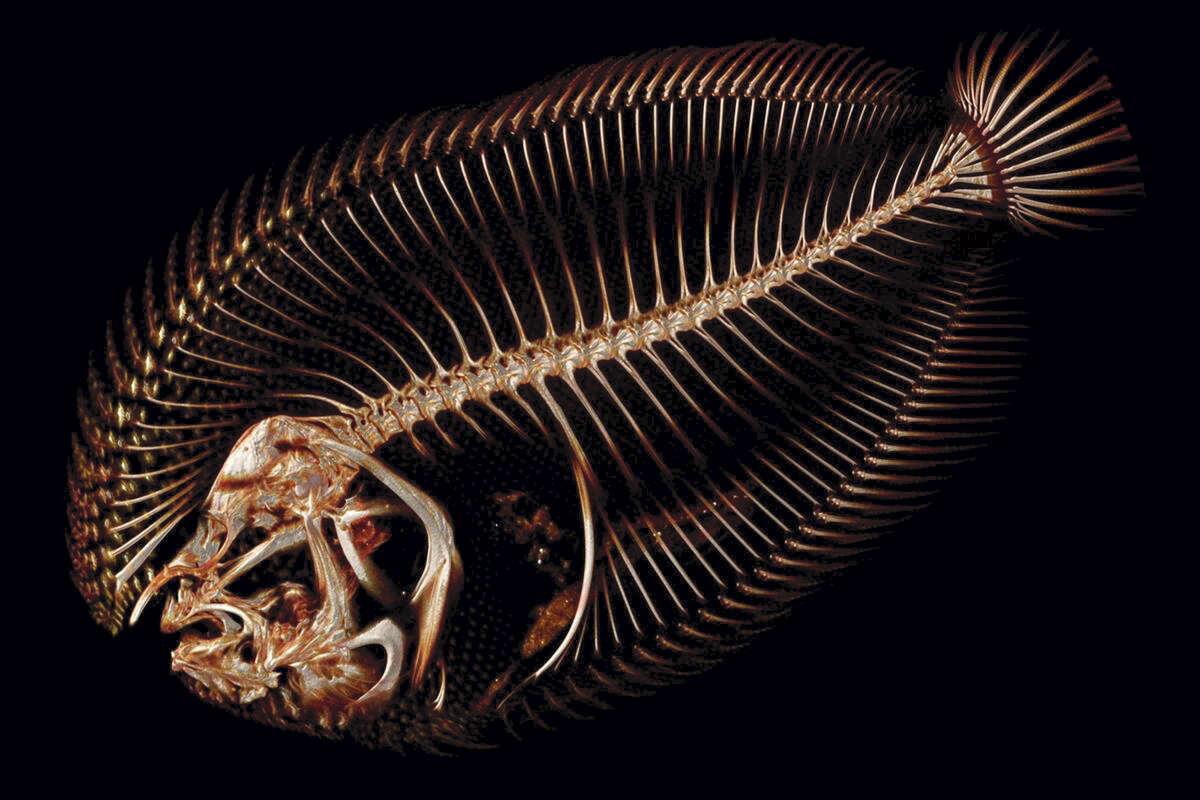This image features an intricately detailed fish skeleton set against a stark black background. Positioned with its head in the lower left corner and its tail extending towards the upper right, the skeleton appears to be upside down. The tail bones fan out gracefully and exhibit a light tan hue, contrasting with the many ribs that prominently display along the spine. The fish's head, which has a mixture of white and brown bones, includes a distinctive curled hook near the mouth area. Surrounding the skeleton, a golden blur with numerous lines envelops the fish, adding a shimmering depth to the composition.